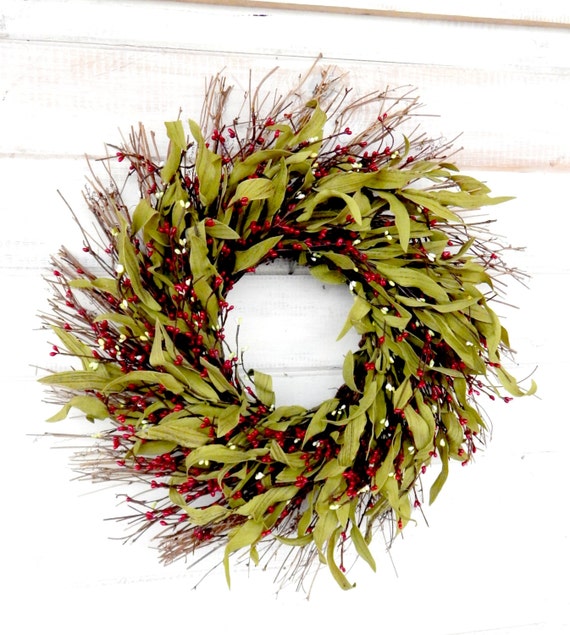This image depicts a Christmas wreath mounted on a white wooden shiplap wall. The wreath is primarily made of long green leaves resembling cornstalks, giving it a somewhat unorthodox yet rustic charm. Intertwined with these leaves are spindly twigs and branches adorned with small red berries, evoking a festive clash of red and green typical of the holiday season. Adding to its texture are hay-like bristles and occasional white artificial flowers, enhancing its rustic appeal. The wreath's overall look is circular and appears spiky, suggesting a rough texture rather than a soft one. The colors—green, red, white, and brown—blend harmoniously, offering an updated take on the traditional Christmas wreath. There is no text in the photo.